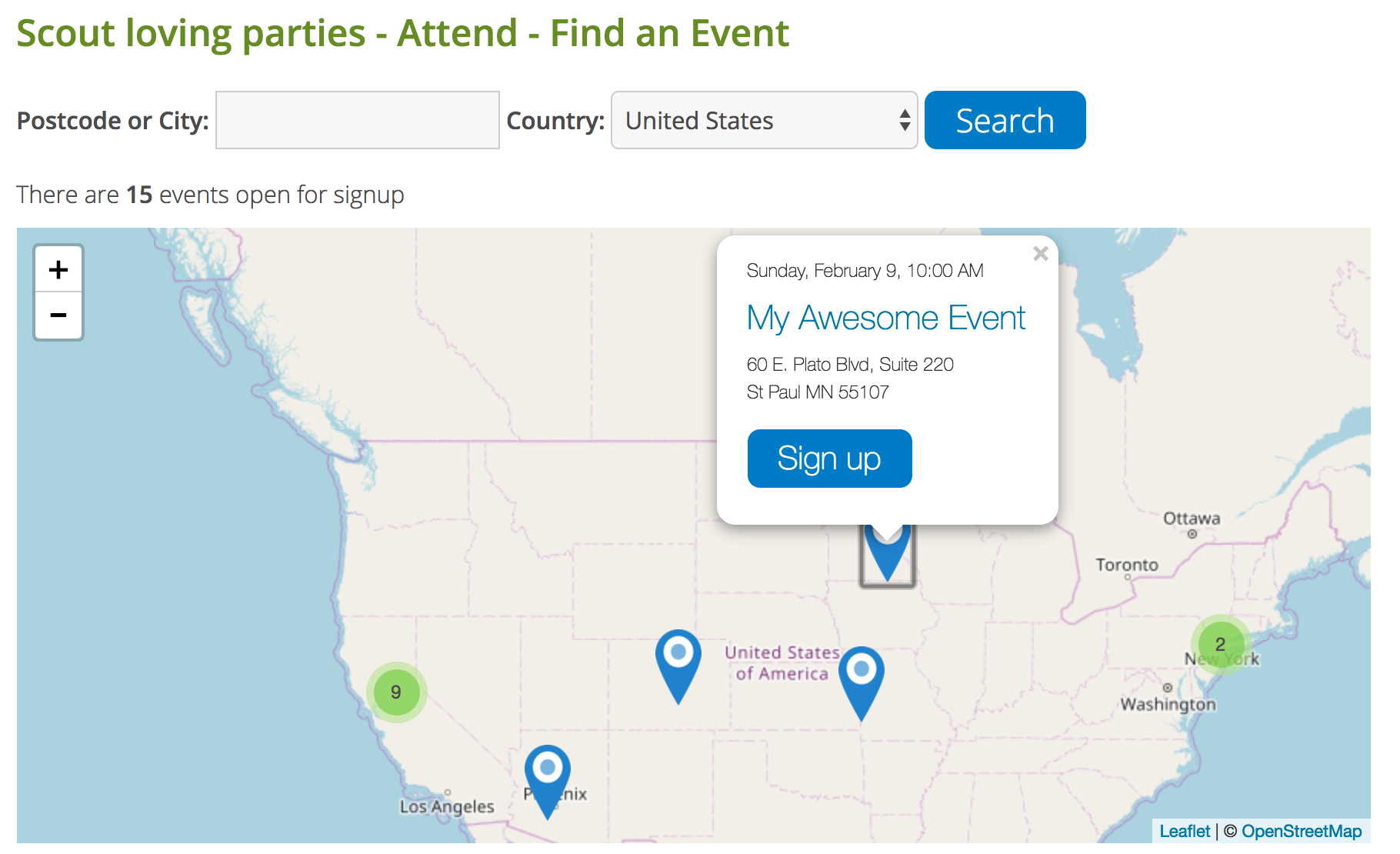The landscape-oriented image features an event search interface for "Scout Loving Parties" prominently displayed in green, bold letters in the top left corner, with the tagline "Attend - Find an Event." Directly below, the subtitle "Postcodal City" appears in smaller yet bold black text, followed by a country selection field defaulting to "United States." Adjacent to this field is a blue "Search" button, inscribed in white.

Beneath this section, a notice on the left informs users of 15 available events for signup. The main portion of the image showcases a detailed map of the United States, extending to major parts of North America. Key geographical labels include "Los Angeles," "Phoenix," "United States of America," "Toronto," "Ottawa," "Washington," and "New York." Notable markers on the map include:
- A green circle with the number "2" over New York.
- Multiple blue location markers flanking the "United States of America" label, one near Phoenix.
- A green circle with "9" on the west coast, unassigned to any specific label.

In the top left corner of the map, there are plus and minus buttons for zooming in and out, vertically arranged with the plus button above the minus button.

Additionally, there is a pop-up box on the map indicating an event:
- Title: "Sunday, February the 9th, 10 a.m., my awesome events" in blue, bold text.
- Location: "60 E. Plato Boulevard, Suite 220, St. Paul, Minnesota, 55107"
- Signup option: A blue rectangular "Sign Up" button.

This pop-up is anchored to a blue location marker on the map, with a small arrow at the bottom of the box pointing towards its corresponding location.